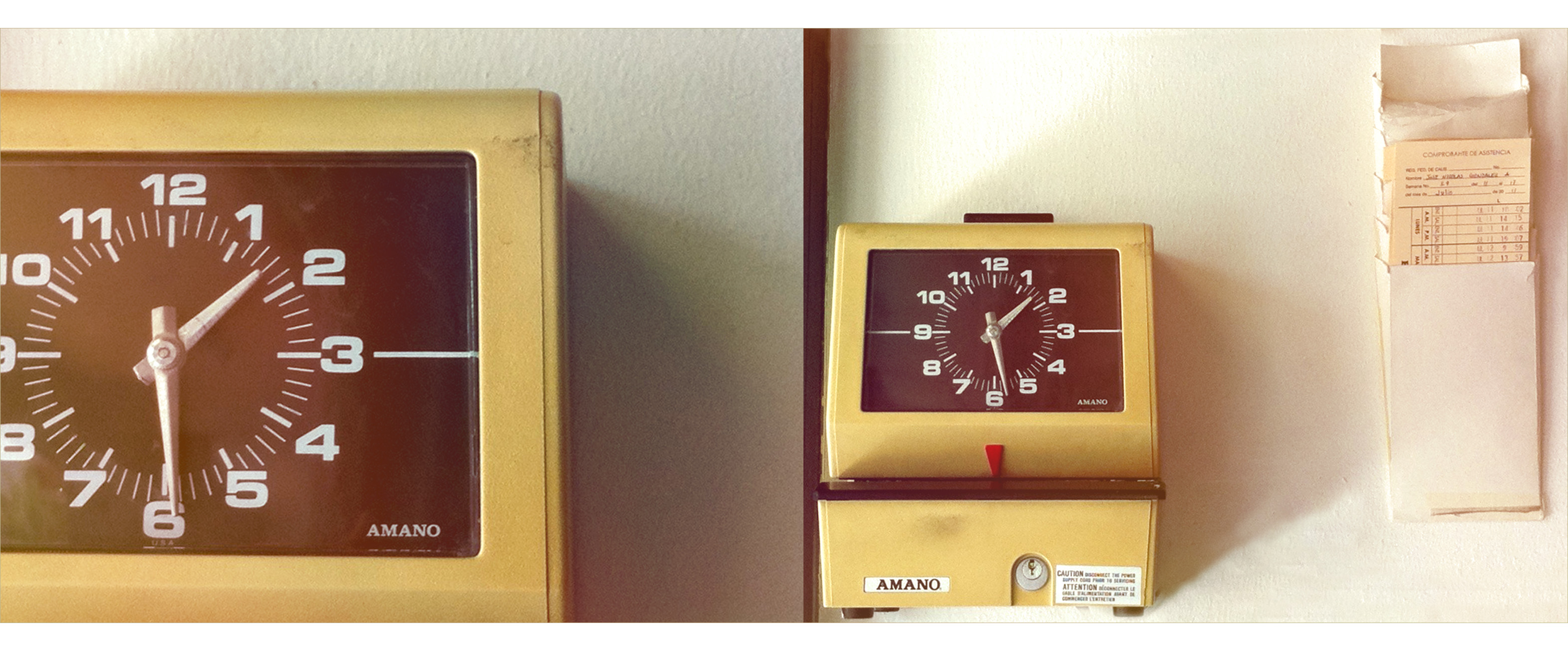The photograph captures a narrow indoor setting featuring two golden-colored clocks with black faces and white numerals (1 through 12) and markers for minutes and hours. Both clocks bear the label "Amano" (A-M-A-N-O) on their dials. The larger clock on the left, showing the time as 1:30, is mounted on a grey wall segment that transitions into white. Adjacent to it on the white wall, the smaller clock, which serves as an old analog timekeeping device for punching time cards, includes a black button, a slit for inserting cards, and a silver keyhole. Attached to the wall on the far upper right is a white holder containing time cards, presumably used by employees to record their work hours. The combination of these elements suggests a typical workplace timekeeping setup.